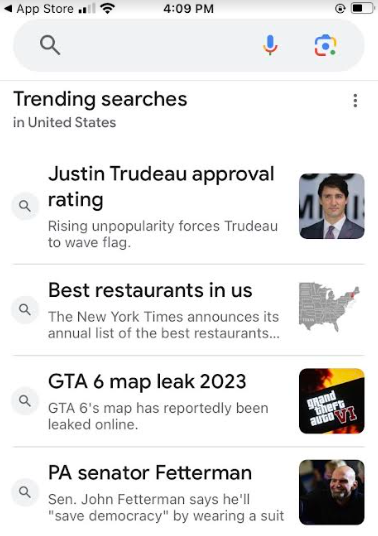This screenshot, likely taken from a mobile phone, showcases a series of trending searches. The time displayed in the center at the top of the screen is 4:09 PM, and to the right, the battery symbol shows a charge slightly less than half full. Prominently at the top is a Google search bar, identifiable by its characteristic blue, yellow, red, and green color scheme, along with microphone and camera icons on the right side. It appears that the search bar has been activated, possibly being the home screen of the Google app, revealing several trending searches below.

The listed trending searches are as follows:
1. **True-to-Approval Rating**
2. **Best Restaurants in the US**  
   - Accompanied by a description: "The New York Times announces its annual list of the best restaurants."
3. **GTA 6 Map Leak 2023**  
   - With the detail: "GTA 6's map has reportedly been leaked online."
4. **PA Center Fetterman**

The layout provides a quick snapshot of current interests and popular topics, reflecting real-time search trends.